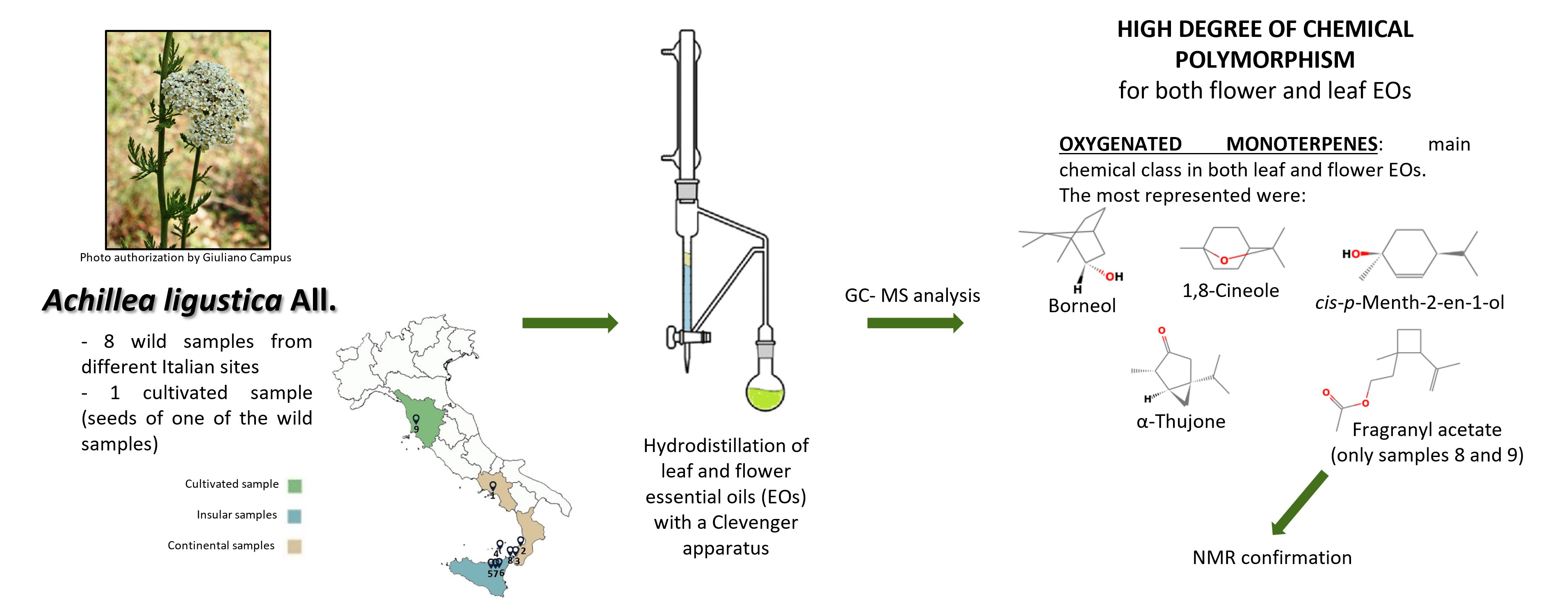A detailed scientific image featuring three sections against a white background. The left section displays a small horizontal rectangular image of a white flower labeled with its Latin name, *Achillea ligustica*. Below it, there is a map of Italy, indicating its cultivation sites, with text stating "eight wild samples from different Italian sites; one cultivated sample from seeds of one of the wild samples." 

A green arrow points to the middle section, which is a technical drawing depicting the hydro distillation process of leaf and flower essential oils using a Clevenger apparatus, with the explanation "Hydro distillation of leaf and flower essential oils (EOs) with a Clevenger apparatus" in black letters.

Another green arrow leads to the final section, which features the text "High degree of chemical polymorphism for both flower and leaf EOs" at the top. Below, it states, "Oxygenated monoterpenes as the major chemical class in both leaf and flower EOs," with specific compounds such as borneol, cineole, and cis-p-menth-2-en-1-ol listed. The section also displays molecular diagrams, primarily hexagonal in shape, illustrating the chemical structure of these compounds.